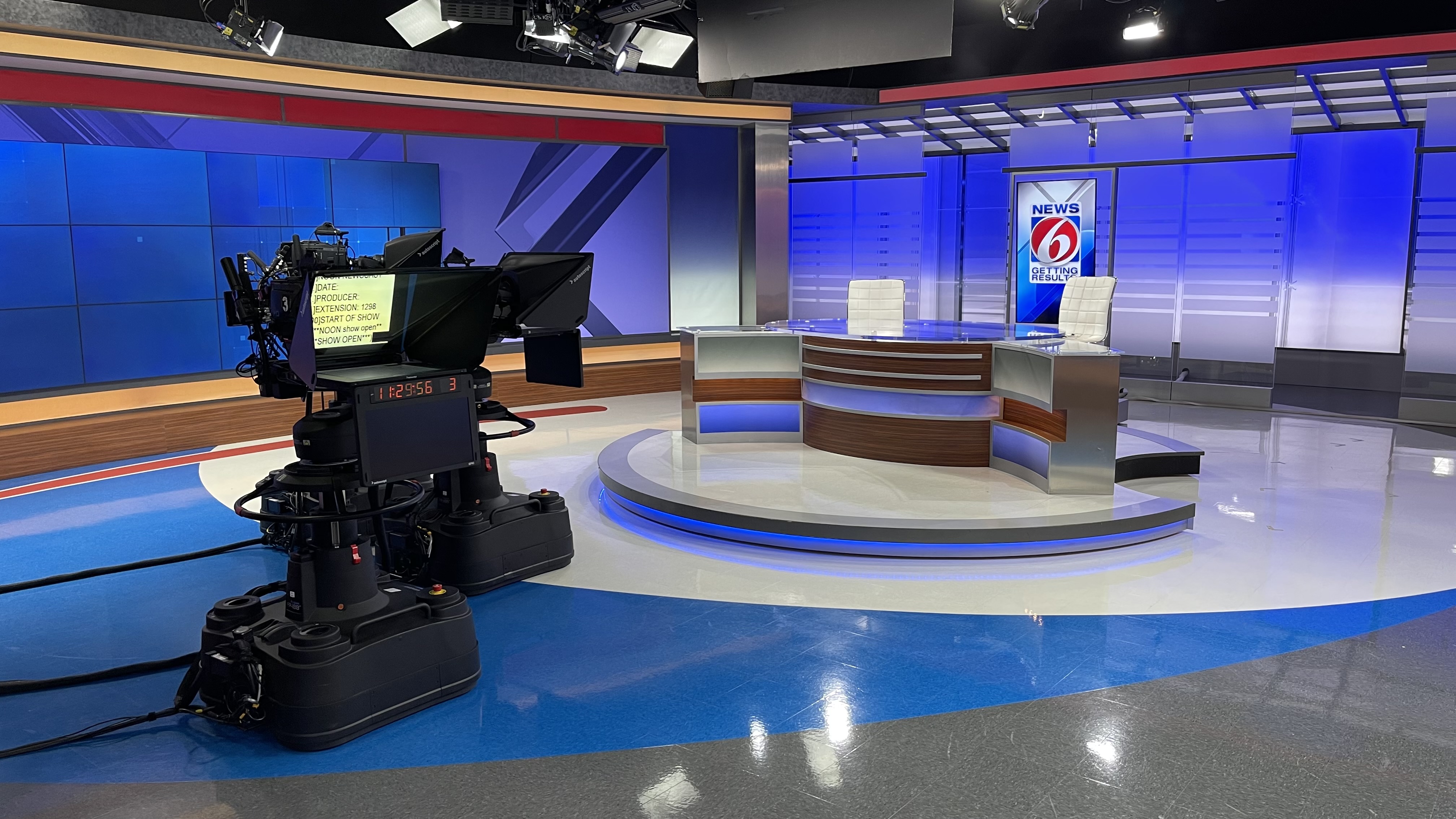This is a detailed photo of an empty, high-tech newsroom studio, typically used for delivering morning or evening news broadcasts. Dominating the background is a large, modern display screen with a blue gradient that prominently features the News 6 logo — a distinctive white number 6 set against a red circle, with the tagline "Getting Results" beneath it. The center of the studio is defined by an arc-shaped, silver desk with wood paneling, accompanied by two white swivel chairs positioned for the news anchors.

On the left side of the image, there is a substantial black camera setup equipped with various recording and teleprompting equipment. A taped yellow paper note on the camera lists stage directions, reading: "Date, Producer, Extension 1298, Start of Show, Noon Show Open, Show Open." Additionally, digital readouts on the camera display the numbers 11-29-56-3, possibly indicating specific timing or settings.

The studio's color scheme mainly features shades of blue, black, and gray, contributing to a sleek, modern atmosphere. Overhead, special lighting rigs are visible, enhancing the studio’s professional appearance. The newsroom is meticulously designed to facilitate smooth operation and effective delivery of news broadcasts.